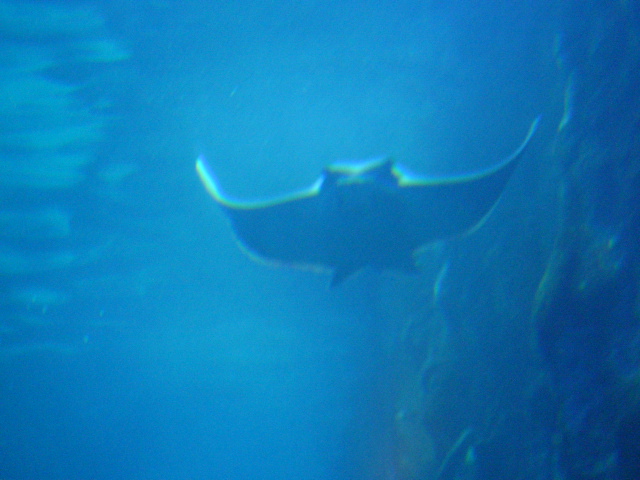Captured underwater, the image features a somewhat grainy, blurry scene likely taken with a less-than-ideal camera. The water is primarily a teal color, gradually darkening from left to right. Dominating the center of the frame is a ray—potentially a stingray or manta ray—swimming directly towards the viewer. The ray spans from roughly 30% to 80% horizontally and from about 50% to 70% vertically within the image. The photograph appears to be taken from a position slightly beneath the ray, indicating that the camera operator was underwater. The right side of the picture is notably darker, making it challenging to discern details in that area. The overall composition suggests that the shore or surface is relatively close.